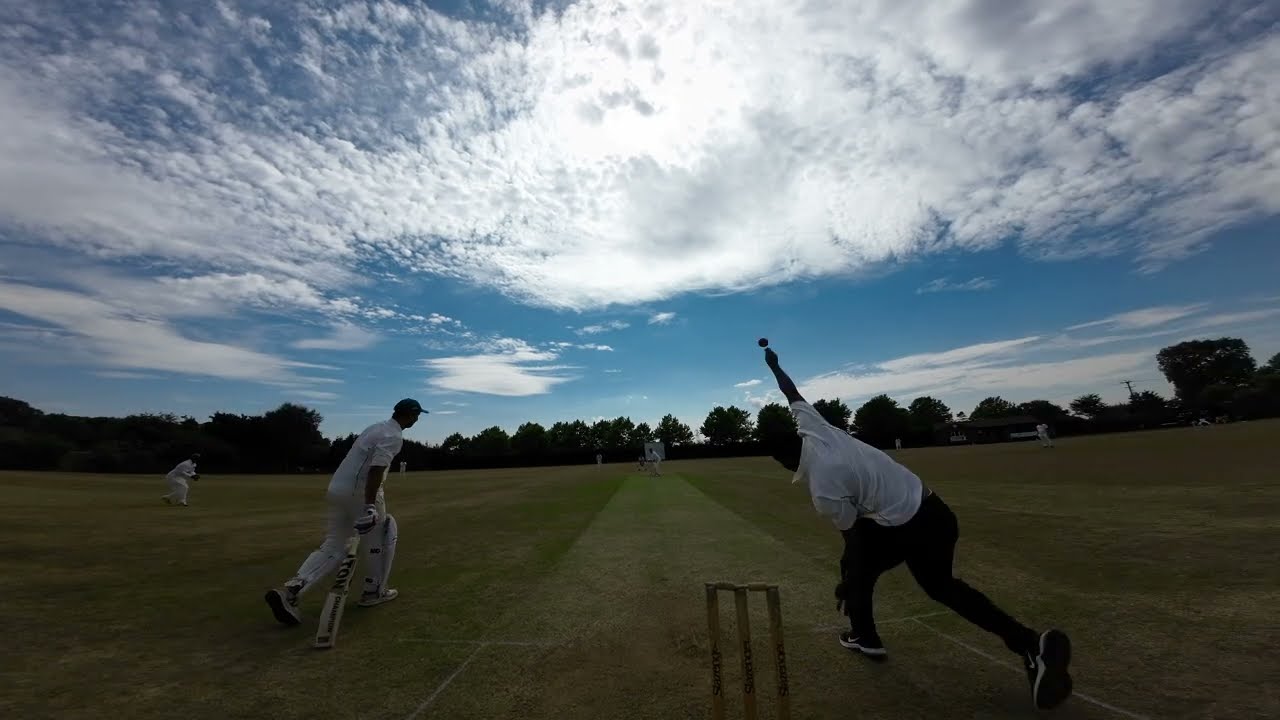This horizontally aligned rectangular picture captures the intense moment of a cricket match played on a vivid green field at ground level. Dominating the top half of the image is a partially cloudy sky with a bright blue backdrop and feathery, white clouds especially concentrated in the upper left-hand side. The sun is hidden behind these clouds. In the front lower right corner, a player in a white shirt and black pants is captured mid-action, with his right arm extended upwards as he pitches the cricket ball, while his left leg is in a lunge position. Directly to his left is the wicketkeeper dressed in all white with a dark cap, poised and seemingly ready to catch the ball; the ball can be seen just above his glove. In the distant background, near the center, stands a small, indistinct figure, the batsman, waiting to hit the ball. Separating the vibrant field from the sky is a row of tall green trees, adding depth and a natural boundary to the scene. The field itself has faint white lines visible at the bottom, demarcating the playing area. There are no texts or signs to distract from the scene, allowing the viewer to focus entirely on the cricket match being played on this partly sunny day.